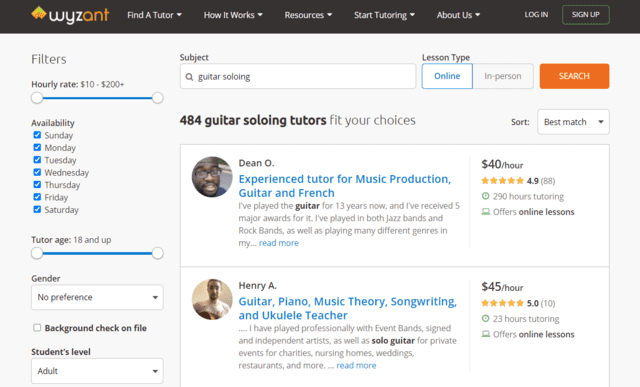This image captures a web page of the Wyzant website, prominently featuring its navigation and search functionalities. The top black border hosts several tabs: "Find a Tutor" (with a drop-down arrow), "How It Works" (with a drop-down arrow), "Resources" (with a drop-down arrow), "Start Tutoring" (with a drop-down arrow), "About Us" (with a drop-down arrow), "Login," and a highlighted black "Sign Up" button.

Below this is a gray filter section to the left, allowing users to narrow their search by hourly rate (ranging from $10 to $200+), and by tutor availability, with blue checkboxes for each day of the week. Additional filters include tutor age (18+), gender (with a drop-down box showing "No Preference"), the option to select only tutors with a background check on file, and the student's level (with a drop-down box currently showing "Adult").

At the top of the search area, there's a subject box filled in with "Guitar Soloing." To its right are buttons for "Lesson Type" (set to "Online" with an option for "In-Person") and an orange "Search" button.

Directly below, a section announces "492 Guitar Soloing Tutors fit your choices," accompanied by a sort box defaulted to "Best Match." 

Following this, two tutor profiles are displayed. The first tutor, Dean O., offers tutoring in music production, guitar, and French. He appears to be African, charges $40 per hour, boasts a rating of 4.9 stars from 88 reviews, has logged 290 hours of tutoring, and provides online sessions.

The second tutor, Henry A., specializes in guitar, piano, music theory, songwriting, and ukulele instruction. He appears to be of European descent, charges $45 per hour, holds a perfect 5-star rating from 10 reviews, has 23 hours of tutoring experience, and also offers online lessons.